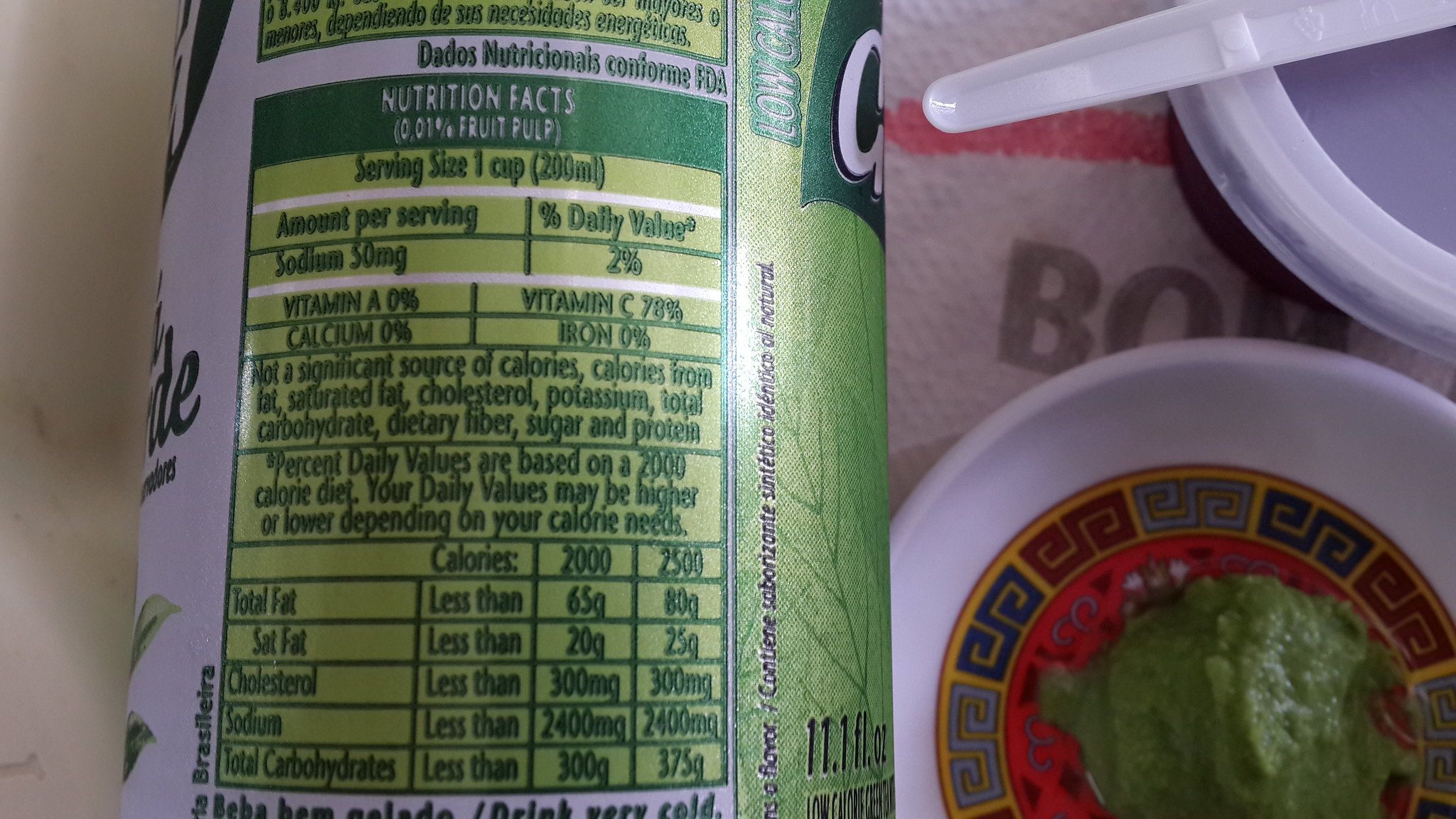A detailed close-up of a nutrition facts panel on the side of a green and white can. The left side of the can is visible with the letters "DE" peeking out, while the right side shows "11.1 full ounces" towards the bottom. The nutrition facts panel is framed with a dark green rectangular border at the top, and a thinner green border along the sides and bottom. The serving size is listed as "1 cup," and the remainder of the panel displays standard nutritional information. In the bottom right corner of the image, there's a small white bowl featuring a Chinese motif at its base, holding a dollop of runny guacamole. The top right corner partially shows a plastic lid for a container and a plastic piece of silverware lying at an angle over a napkin.